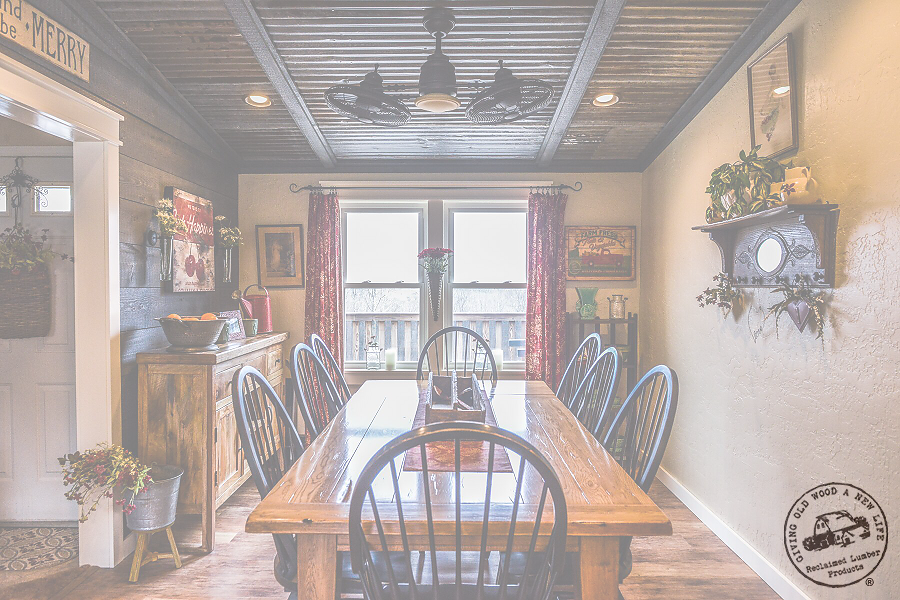This photograph depicts a rustic dining room that exudes a cozy, farmhouse ambiance, accentuated by a hazy or stylistically softened appearance. Central to the room is a large wooden dining table surrounded by eight slatted wooden chairs—three on each side and one at each head. The table features a fabric runner with a decorative box at its center. The back wall is adorned with two large windows flanked by picture frames. Between these windows sits a vibrant bouquet of flowers, adding a pop of color to the scene.

To the left of the windows stands a wooden sideboard displaying an array of items, including a bowl of oranges, a picture frame, and a watering can. Opposite this is another wall decorated with a picture frame and a shelf holding various plants. The room also contains a unique double ceiling fan, where two fans are whimsically suspended from the ceiling, which is accentuated with exposed wooden beams. 

Red patterned curtains frame the windows, adding a touch of warmth with their design, and there's an entryway visible on the left side of the image. The room effectively combines practical elements and decorative touches, featuring reclaimed lumber products that highlight the charm of old wood given new life.